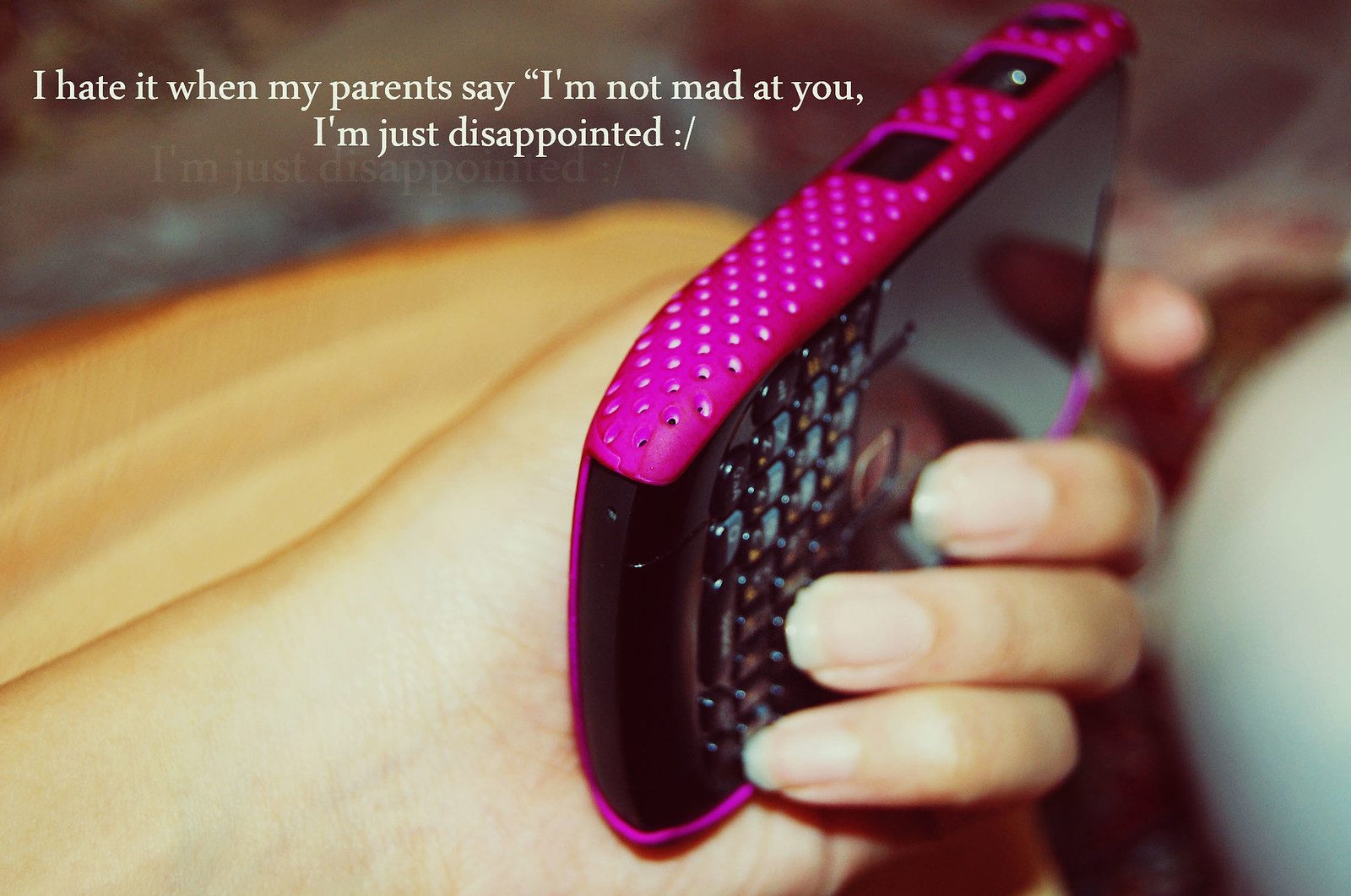A full-color photograph captures a Caucasian girl or woman's hand, judging by the longer fingernails, holding an older style smartphone with a purple and black design, featuring raised buttons instead of a touchscreen. The background is blurred, making it difficult to discern specific details, but there are hints of white and brown blurs on either side. The phone displays a text in small white font at the upper left-hand side that reads: "I hate it when my parents say, 'I'm not mad at you, I'm just disappointed.'" Adding to the sentiment, the phrase repeats faintly below, creating a poignant and relatable digital poster effect.